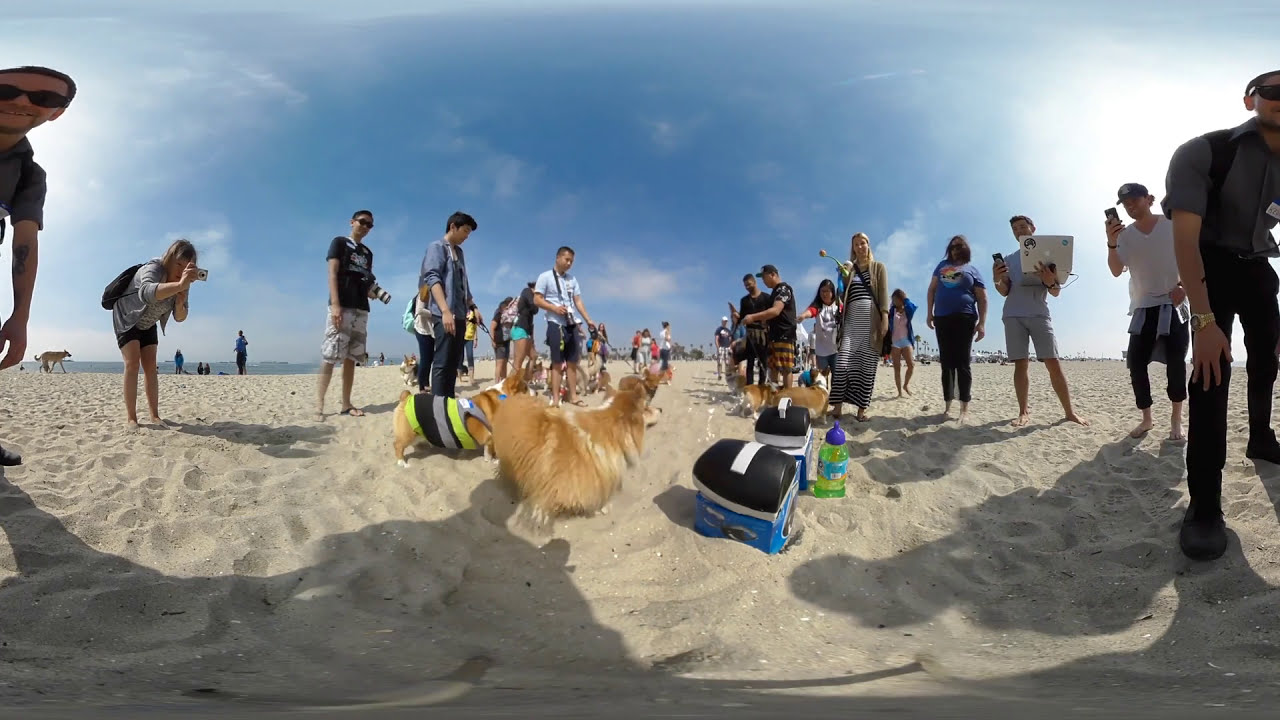The scene is set on a sunny beach under a clear blue sky, where light-colored sand stretches across the ground, covering the entire floor up to halfway through the image. In the center of this detailed, landscape-oriented, panoramic color photograph, a semi-circle of people sparsely gathers, all intently watching and taking pictures of two distinct dogs. The first dog, positioned centrally, is a fluffy, tan-colored animal with light brown fur, exuding a playful aura. To its left stands a short, somewhat chubby dog clad in a striking yellow and black striped jacket.

Amidst the crowd, notable individuals include a woman leaning over at the waist with a camera poised to capture a perfect shot, a young man with dark hair in a black t-shirt and white swim shorts wearing sunglasses, and another man in a white t-shirt and black shorts also with a cell phone. A gentleman with a blue shirt and jeans stands nearby, while a man with sunglasses, a camera hanging from his neck, is observed next to a woman in a blue shirt among others.

Scattered around the scene, several coolers can be spotted: a prominent blue one with a black lid in the foreground, accompanied by a green water bottle, and other coolers close by. All these elements combine to create a vivid and lively depiction of a collective moment enjoyed on a beach, captured in rich detail with a photographic realism that highlights the joy and spontaneity of a shared experience in a natural setting.